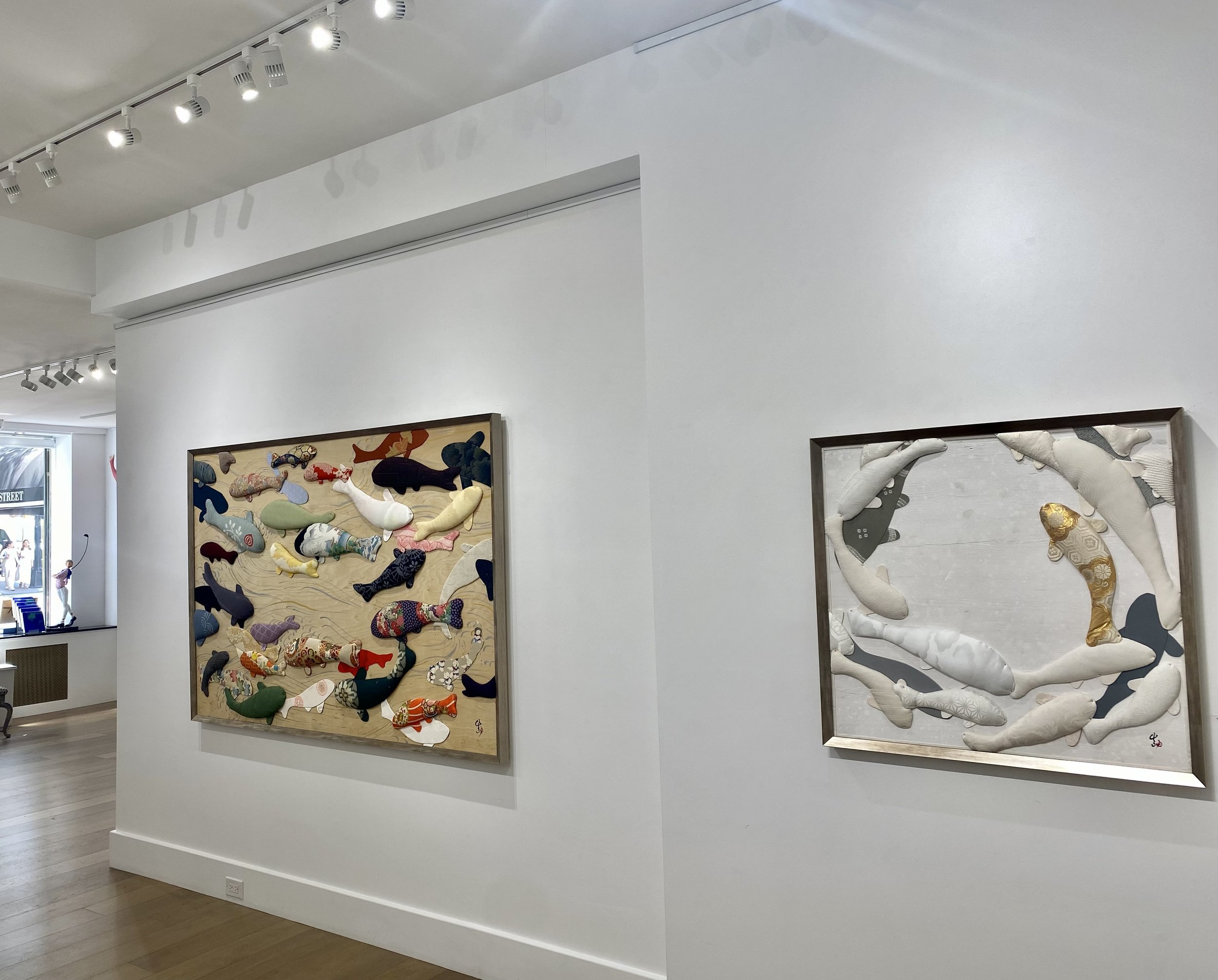The image captures an art display on a stark white wall, possibly in a modern home or an art gallery. On the left side of the wall is a large canvas print with a textured, 3D motif of multicolored fish—including hues of orange, dark green, black, red, purple, gray, and white—swimming against a tan, muddy-looking background. To the right, another art piece, smaller and encased in a sleek silver frame, features a similar 3D fish motif. In this piece, the fish are primarily shades of white, with a few gray ones, a blue one, and a distinctive single gold fish with a shiny appearance, all swimming in a circular pattern against a white plaster background. The light wood-planked floor is visible in the bottom left, anchoring the scene, while the track lighting in the top left illuminates the detailed artwork, providing a cohesive and vibrant artistic display.